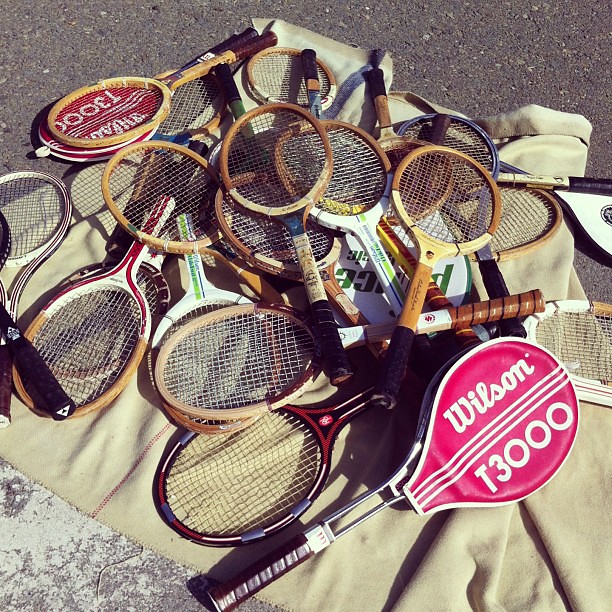In this photograph, we see a jumble of vintage racquetball and tennis racquets, predominantly made of light wood, all piled on top of one another. They rest on a beige or gray blanket spread out on a black cement path or asphalt, possibly part of a tennis court or parking lot. Most racquets feature wooden heads with light-colored mesh centers, and many handles are wrapped in black tape, although some have brown grips.

A standout among the collection is a more modern racquet with a red cover adorned with the text "Wilson T3000" in white. This particular racquet has a silver body and a handle wrapped in dark brown tape. Additionally, one racquet displays a green stripe running along its handle. Various racquet covers are partially visible beneath the pile, adding to the impression that these racquets were hastily gathered together, perhaps by a team after a match.